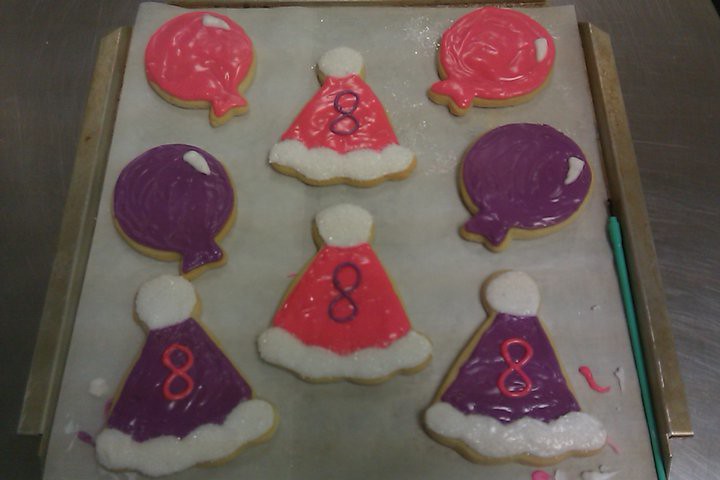This is a detailed photograph of a tray showcasing eight festively decorated cookies, meticulously placed on a white wax sheet that covers a metallic gray baking sheet. The cookies are grouped into two distinct shapes and color themes, each presented as a delightful visual treat. 

Positioned in the pattern of three on the left, three on the right, and two in the center, the arrangement features four cookies shaped like balloons or water balloons with nozzles at the ends. These balloon-shaped cookies come in bright pink or purple hues, each adorned with a small white stripe of frosting that adds a touch of definition and charm.

The other four cookies take the form of Santa Claus hats. Each hat is meticulously iced with either pink or purple frosting, and they feature a '8' piped in contrasting colors—pink on purple hats and purple on pink hats. The Santa hat cookies are further embellished with a white frosted trim at the base and a small white circle at the tip, mimicking the traditional fluffy details of a Christmas hat.

In the background, the setting reveals a steel-colored surface, potentially another metallic platter, enhancing the festive feel of the overall composition. A glimpse of a teal stick can be spotted on the right, adding an additional touch of color to the scene. This detailed and vibrant arrangement captures the essence of holiday cheer and skilled baking artistry.